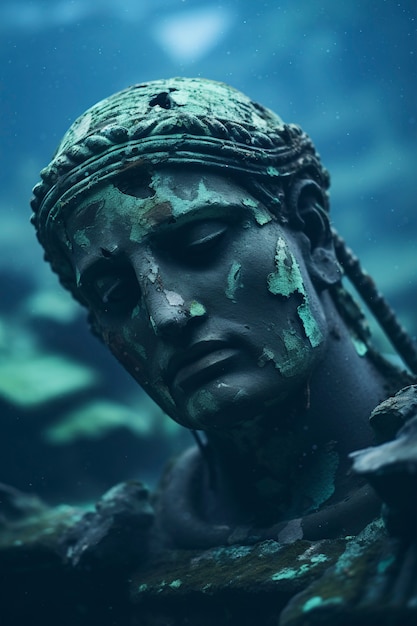This portrait-shaped image features a very weathered statue of a figure whose identity and gender are ambiguous. The statue depicts a bust with the head and shoulders visible, showing a dark green facade with light green flecks, suggesting significant weathering. The face of the statue, turned downward towards the lower right corner of the image, exudes a sad and contemplative expression, accentuated by the drooping corners of the mouth and almost closed eyes. Adding to the statue's solemn look is a braiding or headdress-like ornamentation around the forehead, intricately tied over the left ear with some strands hanging down. Despite the initial ambiguity about whether the green comes from a filter or oxidized copper, the statue's worn appearance and green hues give it an eerie, almost melting look. The background is a blurred mix of dark blue and light green, possibly resembling sky or stone with moss, further emphasizing the ancient and deteriorated essence of the statue.